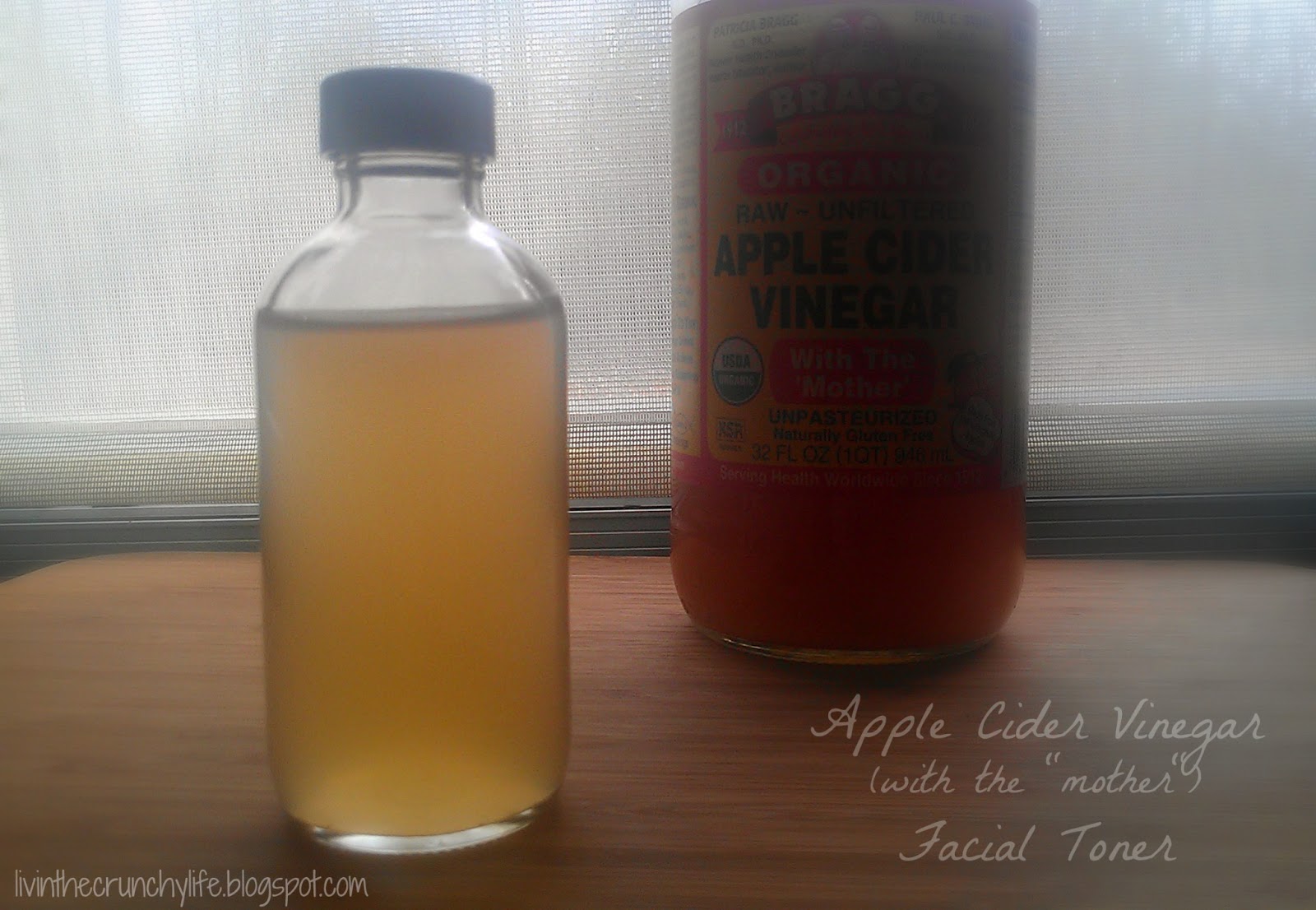This detailed and descriptive caption synthesizes the key repeated elements and details from each caption provided:

"In this close-up, slightly blurry image, a clear plastic bottle with a blue cap sits on a brown wooden table, containing what appears to be apple cider vinegar. To the right of this small bottle is a larger, orangey bottle labeled 'organic apple cider vinegar,' with the words 'apple cider vinegar with the mother facial toner' written in cursive on the right side of the image. A window with a mesh-type shade serves as the background. In the bottom left corner of the photo, a website in white font reads: liveinthecrunchylife.blogspot.com."